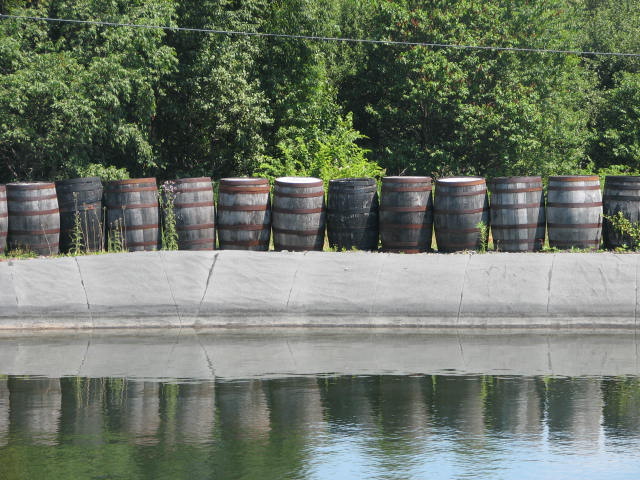The image showcases a small cement bridge spanning over blue and gray water, which reflects the structures above. Positioned centrally on this cement surface are 12 well-weathered gray barrels with rusted steel hoops, arranged in a straight line from left to right. These barrels are mirrored in the water below. Behind the barrels, a dense area of tall trees with vibrant green foliage dominates the background, with shades ranging from solid green to nearly black due to the varying light conditions. A wire, possibly an electrical or telephone line, stretches across the very top of the image, hinting at a man-made presence amidst the natural setting. The scene, captured in square format, exudes a serene, outdoor ambiance on a bright, sunny day.